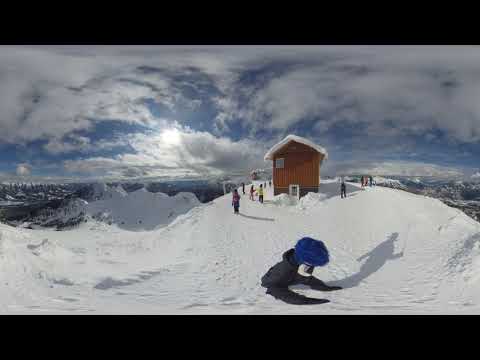This landscape-oriented color photograph captures a panoramic winter scene with a distinct separation between the snowy foreground and the vibrant sky. Dominating the bottom half of the image is a snow-covered slope, rolling gently from left to right and dotted with some dark, stick-like forms that may be distant trees. In the middle ground, a small brown wooden structure, likely a hut or cabin, stands covered in snow with a group of people milling around it. This building features a snow-laden roof and what appears to be a white door. 

In the foreground, on the right, a person dressed in a black snowsuit and a blue helmet or hat is seated in the snow, holding a selfie camera. The top half of the image showcases a strikingly blue sky filled with variously patterned clouds, with the sun peeking through some darker patches. In the distance on the right, there is a panoramic view of a red two-story building, also covered with snow, reinforcing the sense of a wintry landscape. This photograph, with its careful composition and representational style, vividly captures the serene yet lively atmosphere of a snowy mountain setting.